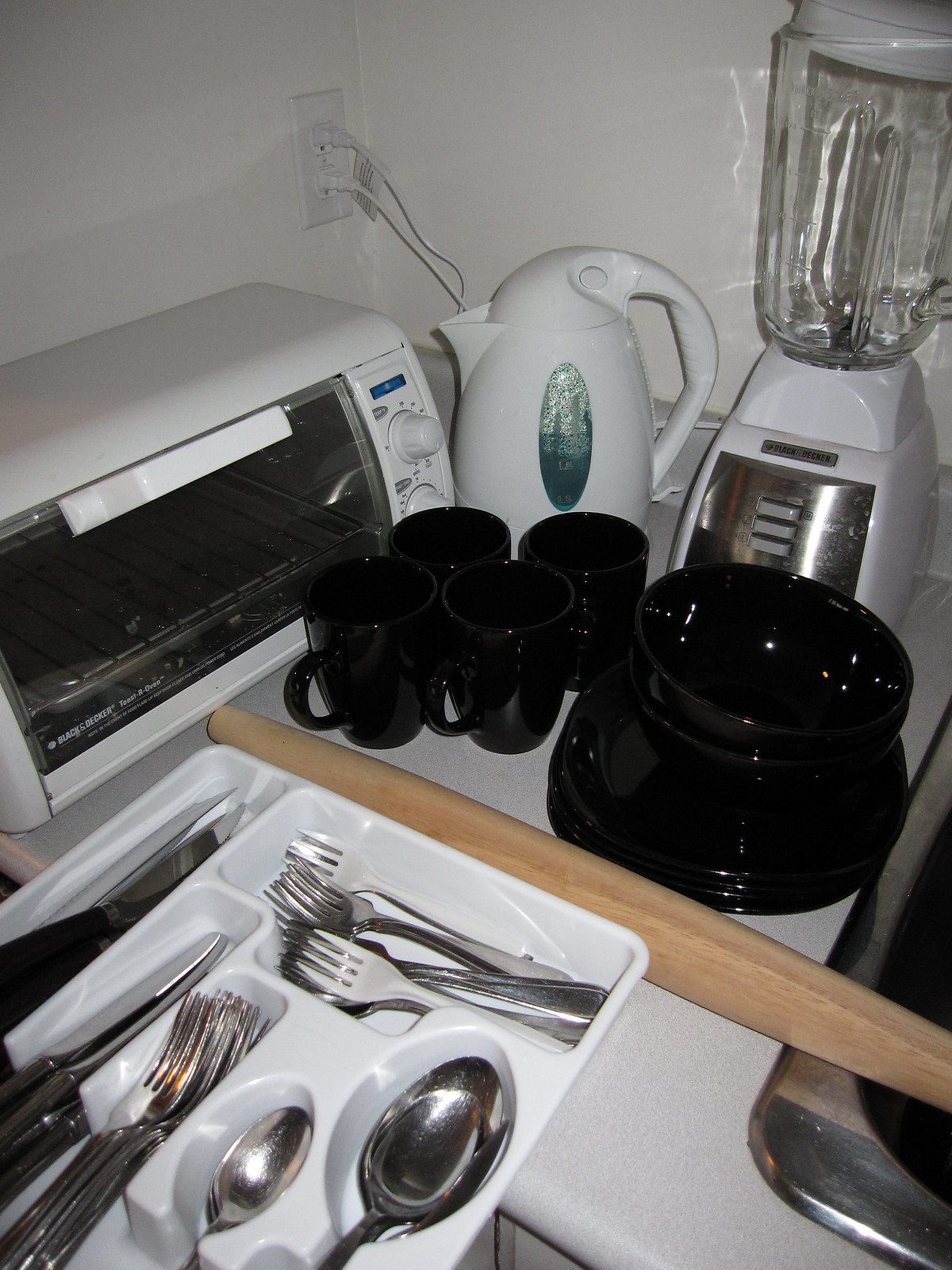The image depicts a kitchen countertop set against a white wall. On the countertop, starting from the top right, there is a blender. The blender has a glass jar with a handle and a white lid, attached to a white base featuring a metal face with gray buttons. Next to the blender sits a white electric teapot with a small transparent window showing the water level, plugged into the wall socket that has two outlets. Moving left, there is a compact white toaster oven with one internal rack and a knob on the front for controls. Beside the toaster oven are several black mugs and a black bowl. A wooden handle or a utensil holder is also visible in this area. Below this setup, there is a rack holding an assortment of forks, spoons, and knives. Towards the far right of the image, part of a sink's outer edge is visible, hinting at the kitchen setup's functional layout.